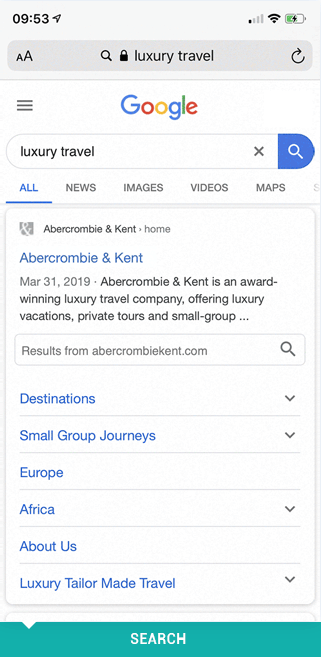**Screenshot of Google Search Results for 'Luxury Travel' on Mobile**

The image is a mobile view screenshot of a Google search conducted in light mode with a white background. The search term entered is "luxury travel", and the category selected is "All". The prominent search result displayed is from Abercrombie & Kent, described as an award-winning luxury travel company offering luxury vacations, private tours, and small group journeys, concluding with an ellipsis.

Below this description, there is an option to view more results from Abercrombie & Kent. Additionally, visible subcategories with dropdown menus include options for "Destinations", "Small Group Journeys", "Africa", and "Luxury Tailor-Made Travel." Notably, the subcategories "Europe" and "About Us" do not feature dropdowns. Towards the bottom, there's another button labeled "Search".

Above the search results, standard Google page navigation options like "News", "Images", "Videos", and "Maps" are visibly unselected. The search bar prominently displays "luxury travel" accompanied by a magnifying glass icon and a lock symbol indicative of secure browsing, positioned under the refresh button.

The screenshot shows that it was captured on a cell phone at 9:43 AM. The device's status bar indicates the battery is approximately half full and charging, the signal is weak but Wi-Fi is enabled.